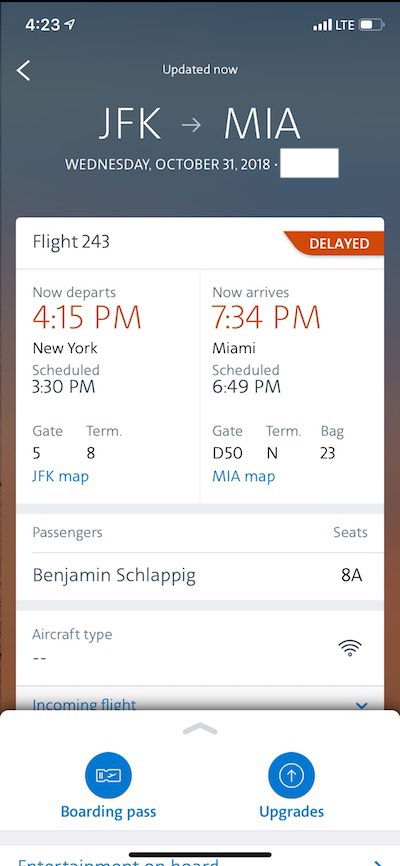The image features a light blue and pinkish background with several flight details prominently displayed. At the top, there’s an arrow pointing upward to the right, next to the number "423". Moving down, there's a leftward-pointing arrow indicating an update: "JFK to MIA, Wednesday, October 31st, 2018".

A large white box dominates the center of the image containing essential flight information. In bold, it reads "Flight 243" with a small red flag indicating the flight is "Delayed". The new departure time is "4:15 PM" with an expected arrival at "7:34 PM". The original schedule has the flight departing New York's JFK at "3:30 PM" and arriving in Miami at "6:49 PM". Gate information specifies: "Gate 5, Terminal 8, JFK" and "Gate D50, Terminal N, MIA" with baggage claim at "Bag 23".

Further details include a blue line separating sections, beneath which there are boxes labeled "Passengers and Seats", listing "Benjamin Schlepping - Seat 8A". Another white box indicates "Aircraft Type" with two small lines beneath, followed by curves that appear to get smaller.

The image also notes an "Incoming Flight" with a downward arrow. Another prominent white box features a blue circle with an upward-pointing square labeled "Boarding Pass" and another blue circle with an upward arrow labeled "Upgrades". A black horizontal line cuts across the layout with a snippet of a blueprint visible at the bottom.

Overall, the image seems to be an informative display of delayed flight details, passenger information, and various amenities or upgrade options.